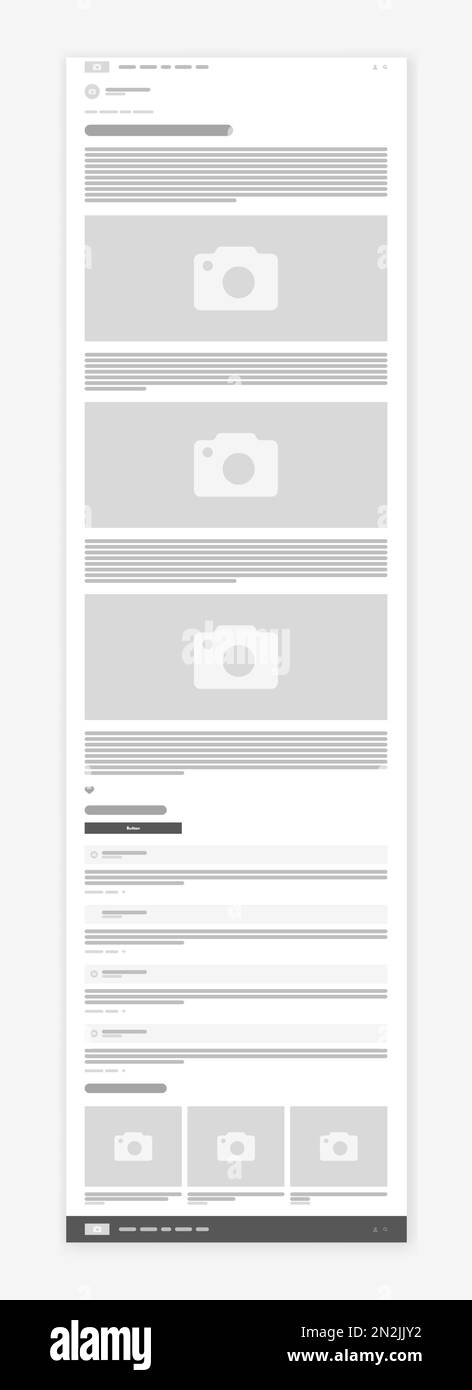This image showcases a detailed website or formatting mock-up on a light gray background. The mock-up features a white page filled with various placeholders indicating where content will be placed. At the top, there's a thick gray rectangle representing the headline area, followed by several thin gray bars indicating the space for a paragraph. Below this, there is a large gray rectangle with a white camera icon, suggesting a placeholder for an image. Further down, the layout alternates between paragraph placeholders and image placeholders. Notably, one of the image placeholders has a watermark that reads "Alami." At the bottom of the image, a prominent black bar spans the width of the layout, featuring the text "Alami" in large white fonts on the left side.